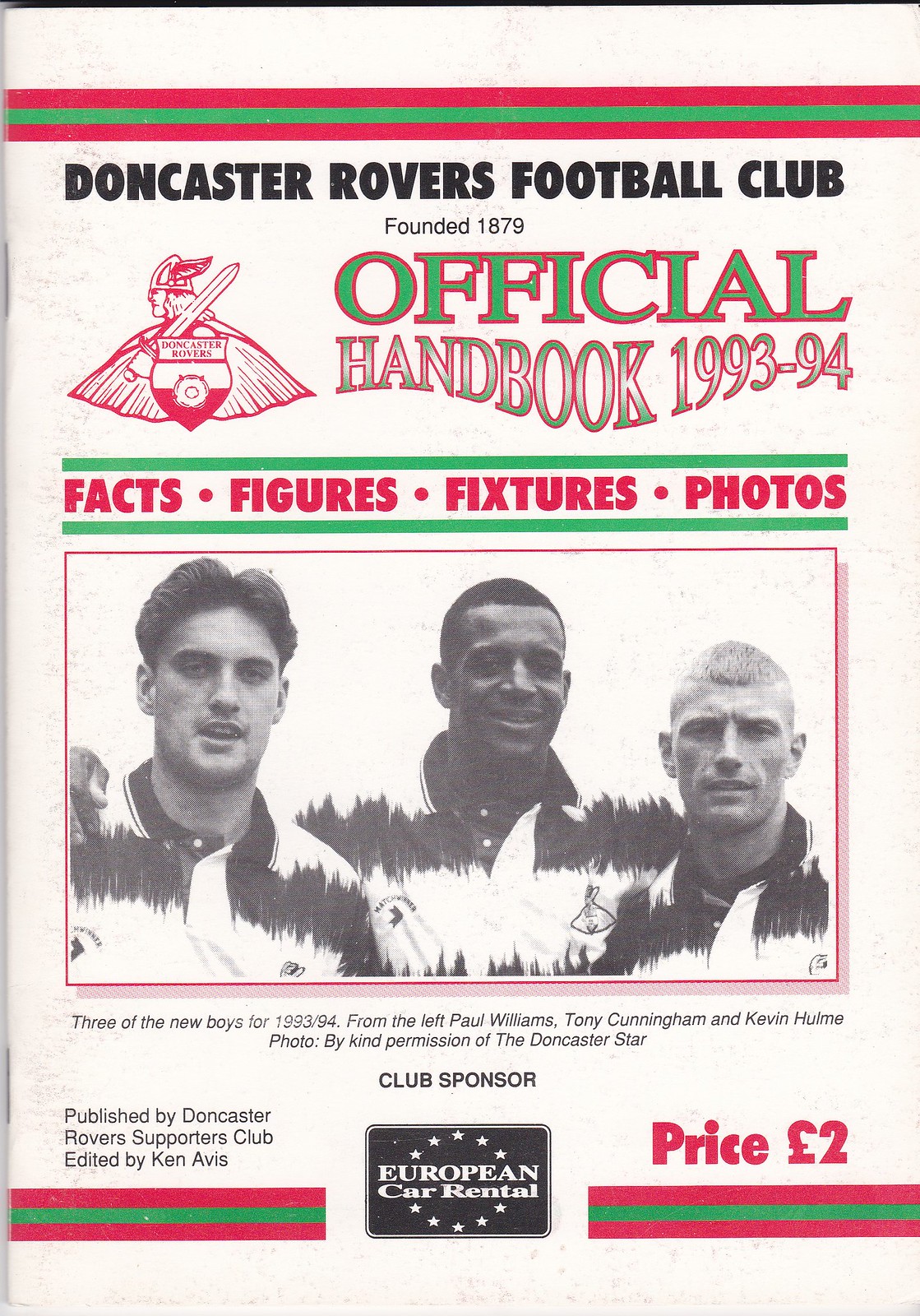The cover of the Doncaster Rovers Football Club’s Official Handbook for the 1993-94 season features a clean white background with three horizontal stripes – red, green, and red – running across the top. Beneath the stripes, the text "Doncaster Rovers Football Club, founded 1879" appears in black. Below this, in green font outlined in red, is the title "Official Handbook 1993-94." To the left of the title is the club's logo: a Viking facing left, with a cape flaring out and a sword resting on his shoulder, wearing a winged conical helmet. The Viking's shield is half white, half red, with "Doncaster Rovers" written in red text on it.

In the center, a black-and-white photo shows three players, identified as Paul Williams, Tony Cunningham, and Kevin Holm, under the caption "Three of the new boys for 1993-94." This photo was provided by the Doncaster Star. Along the bottom of the cover, additional texts include the club sponsor, European Car Rental, on the bottom right, and the price, two euros, on the bottom left. The handbook is published by the Doncaster Rovers Supporters Club and edited by Ken Avis. Just above the photo, the words "Facts, Figures, Fixtures, Photos" are printed in red font between two green lines.